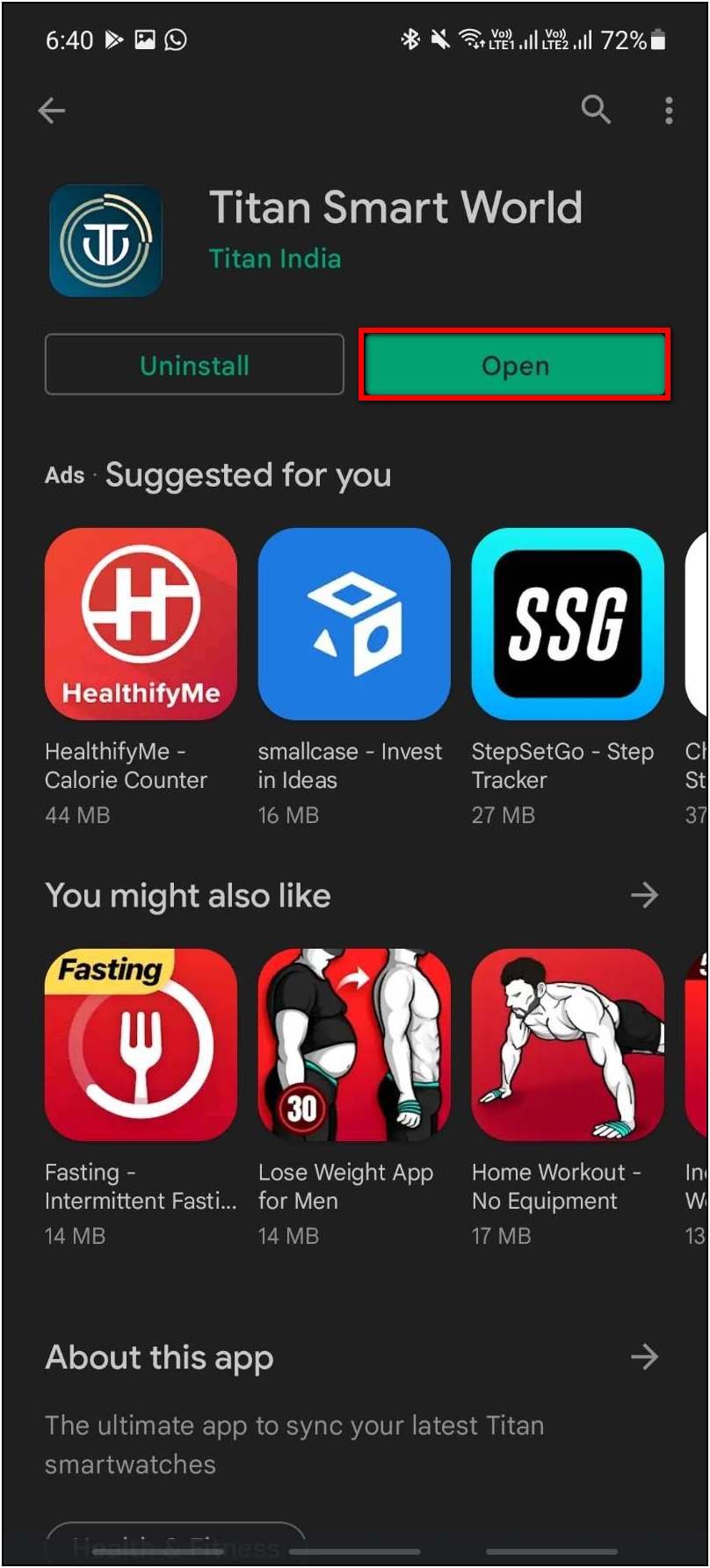This screenshot, captured on a mobile phone (likely an Android device), displays the Google Play Store interface. The screen showcases the app "Titan Smart World," developed by Titan India. Displayed prominently are two primary options: "Uninstall" and "Open," with the "Open" button highlighted in a red box, indicating the app is installed and ready for use. Below this, a section titled "Ads suggested for you" presents recommendations for various health and investing apps. Further down, a "You might like" section suggests additional diet and exercise apps. The "About this app" section describes Titan Smart World as the ultimate application for syncing the latest Titan smartwatches. The entire interface is in dark mode, giving the background a sleek, dark appearance.